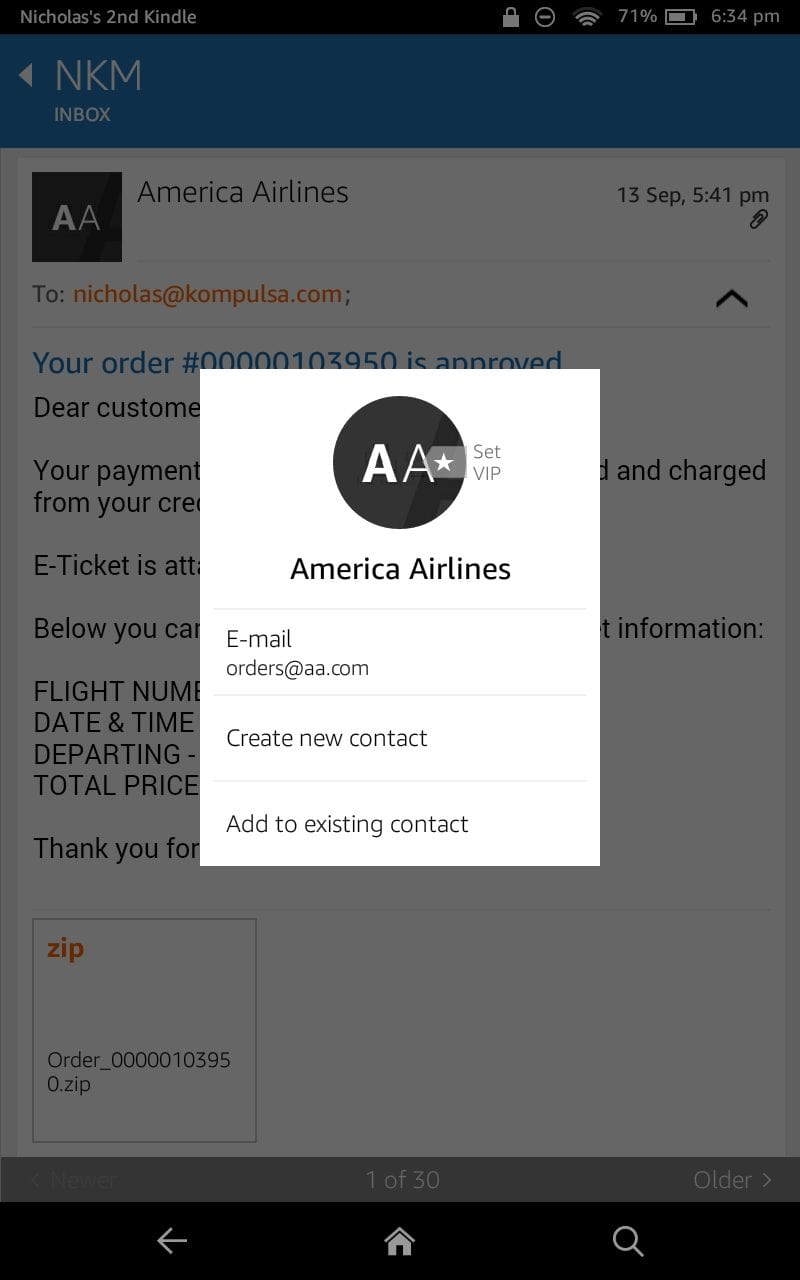The image is a semi-obscured screenshot depicting an email interface on a web page, predominantly from American Airlines. The background showcases an email from America Airlines containing an e-ticket order confirmation, but it is partially obscured by a gray filter, making the text difficult to decipher. In the top left corner, the screen indicates the device name as "Nicholas's Second Kindle," while the top right corner displays a padlock icon, a wireless signal icon, a battery icon showing 71% charge, and the time which reads 6:34 PM.

At the top of the email, it is headed "NKM Inbox," with a timestamp of "13 September, 5:41 PM". The email is addressed to Nicholas at the email "compulsa.com," confirming that order number "00000103950" has been approved. The visible text begins with “Dear customer.”

Superimposed on the email is a white pop-up box containing a circular AA logo with text beneath it reading "Set VIP." Further down, the pop-up displays additional information such as "America Airlines," followed by the email "orders@AA.com" and options to "create new contact" or "add to existing contact."

The pop-up obscures significant parts of the underlying email, making critical details such as the flight number, date and time of departure, departing flight time, and total price unreadable. The legible portion of the email informs the customer about their payment and charge related to the e-ticket, but specific details remain hidden. The email concludes with a thank you note and includes a zip file attachment likely containing further relevant information regarding the booking.